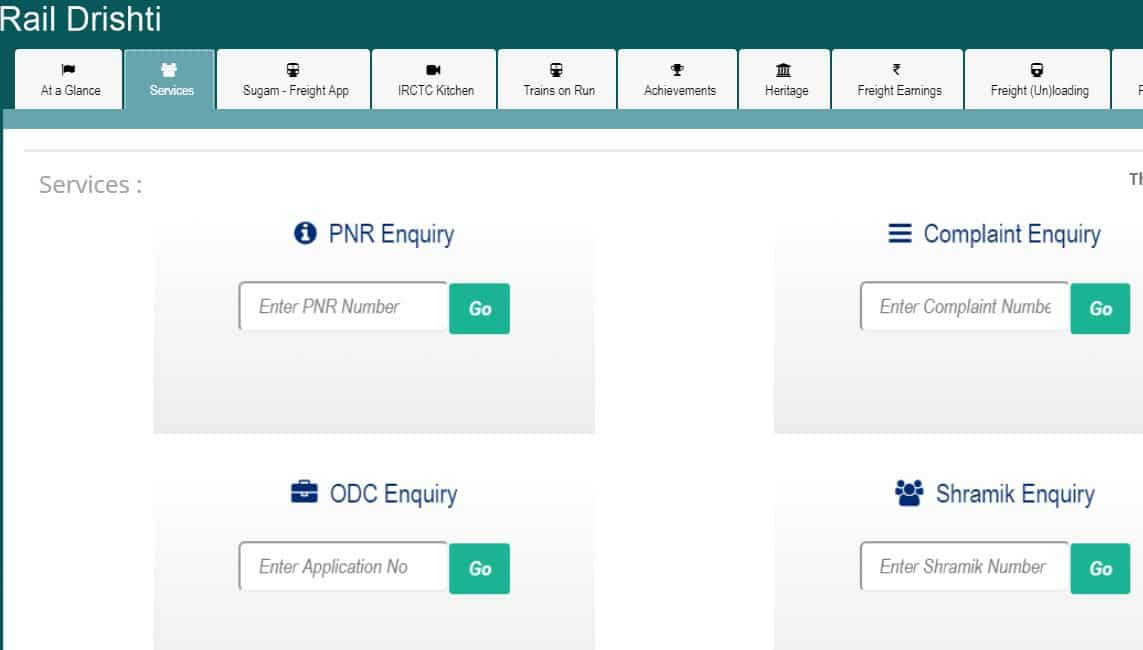The image portrays a computer screen displaying a startup interface for a customer service call, predominantly blank with minimal content. At the very top, there is a dark green header featuring the text "Rail Drishti" in inverted colors. Below the header, several tabs are organized in a row, labeled in the following order: At a Glance, Services, SUGM Freight App, IRCTC Kitchen, Trains on Run, Achievements, Heritage, Freight Earnings, and Freight Unloading. 

The highlighted tab is "Services," revealing four possible inquiries: PNR Inquiry, Complaint Inquiry, ODC Inquiry, and SRAMIC Inquiry. Each inquiry section contains a text box prompting the entry of the relevant number (PNR number, complaint number, ODC number, or SRAMIC number) and a corresponding "Go" button to initiate the inquiry.